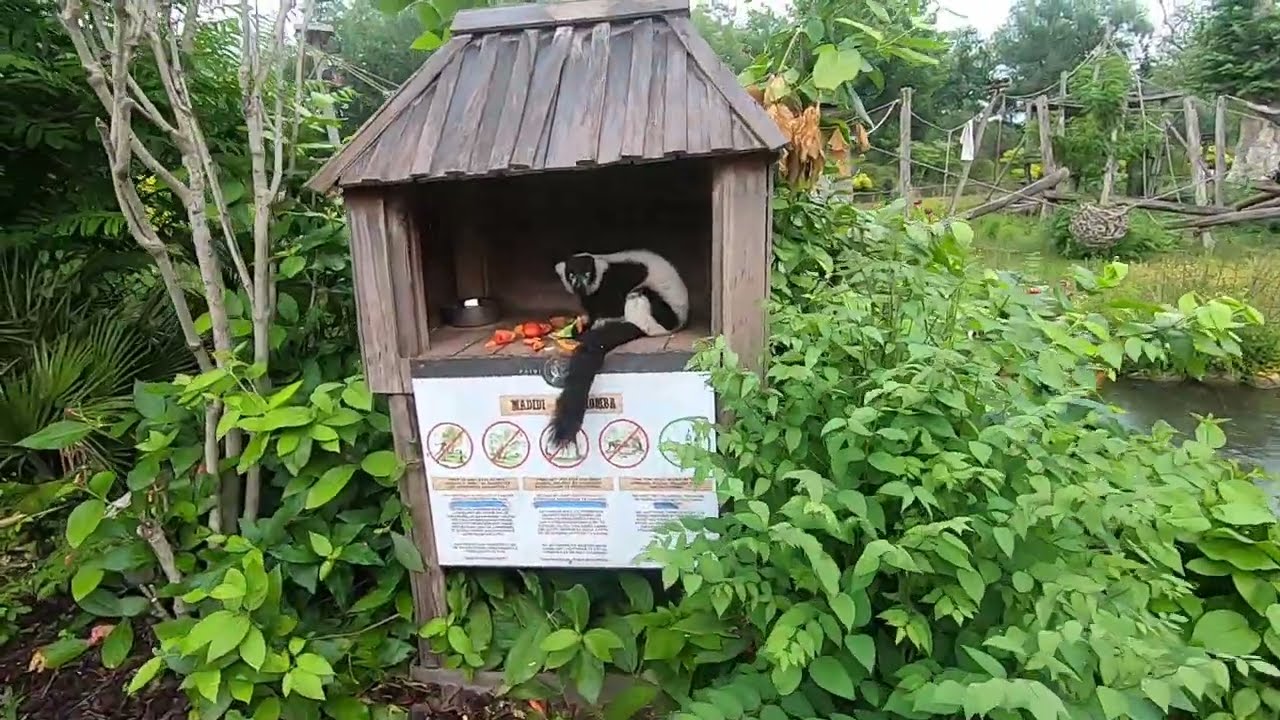Under an overcast sky in a lush, jungle-like zoo enclosure, a small wooden shed occupies the center of the scene, surrounded by dense green foliage and tall, thin tree trunks on the left. The shed, taking up about one-fourth of the view from bottom up, has an enticing array of fresh fruits and vegetables, where a black-and-white lemur enjoys a meal. The lemur, with its distinctive oval-shaped black face, white body, and long, fluffy black tail marked with spots, gazes directly at the viewer. Below the open top half of the shed, a white sign is adorned with unidentifiable text and five circles—four brown, one green—potentially indicating zoo instructions or information about the lemur. In the background, larger leafy plants and an orangey-leafed tree enhance the tropical ambiance. A water feature, possibly a pond, sits in the back right, separating the feeding hut from a complex arrangement of wooden climbing structures connected by ropes, designed to enrich the lemur's habitat. The dense foliage and intricate habitat elements create a naturalistic and engaging environment for the charming creature.